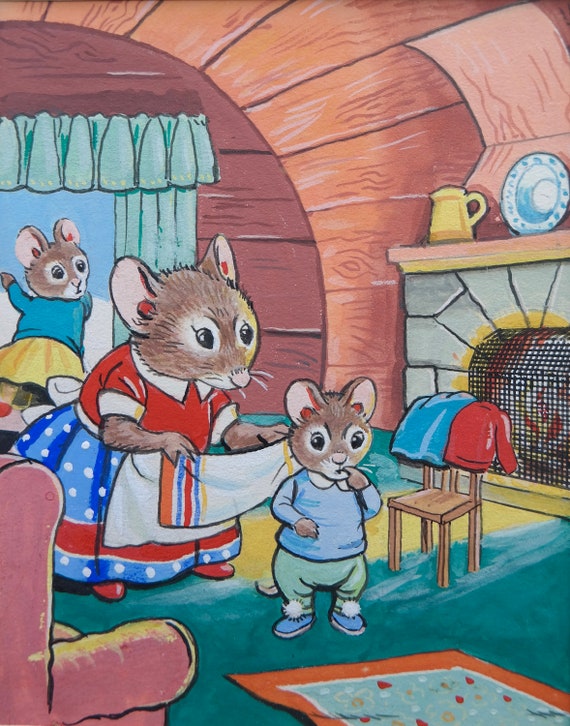This charming hand-drawn cartoon depicts a cozy scene featuring a brown mice family inside a log cabin. The centerpiece is the mother mouse, standing in the middle dressed in a red and blue polka-dot dress with red shoes, holding a towel likely ready to dry one of her children. She has white accents on her collar and sleeves. The baby mouse closest to her, who might be a boy judging by his attire, is wearing green pants, a blue shirt with a big white collar, and blue shoes with white pom-poms. He is looking at something on the floor, which appears to be an orange throw rug on the blue floor. 

The background shows the interior of the cabin with its wooden walls and a sphere-shaped roof. To the left, there is a window framed by teal curtains. A second baby mouse, a little girl wearing a blue sweater and a yellow dress, has her paws on the window frame and has turned her head back towards the rest of the family. 

The homey setup includes an orange carpet, a pink plush chair, and a wooden chair with sweaters draped over its backrest. A warm fireplace sits to the side, with clothes drying on the chair nearby. On the fireplace mantle, a plaque and kettle can be seen, adding to the snug ambiance of the scene. The cabin, bathed in daylight, gives a warm, inviting feel to the family moment captured in this delightful cartoon.